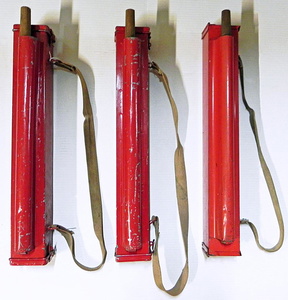This photograph showcases three identical long, narrow, rectangular red metal boxes, each featuring a brown or tan cloth-like carrying strap. These boxes are positioned side by side against a white background, where their shadows are prominently displayed. Each box has a cylindrical holder attached to the front, containing an unidentified wooden object that could potentially be a tool, rod, or instrument component. The metal surface of the boxes has a shiny, slightly worn appearance, indicative of their usage. Despite their purpose being unclear, the detailed arrangement and visible handling straps suggest they are designed for practical use.